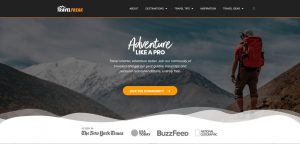This is an annotated screenshot of a travel website's homepage. The website offers travel information and sign-up options. The text and buttons are blurry. At the top, there's a black banner with an indistinguishable white and orange text. It includes five clickable options in the header, their labels unreadable. At the bottom, logos of reputable sources like The New York Times, USA Today, BuzzFeed, and National Geographic are visible. In the middle, there's a bold tagline, "Adventure Like a Pro," with a brief, unreadable description below in white text. There's also an oval-shaped clickable bar with unreadable text. The background image shows a hiker, identified by a red backpack and a hat, standing on a snowy mountaintop, facing away from the camera, with an expansive sky behind.